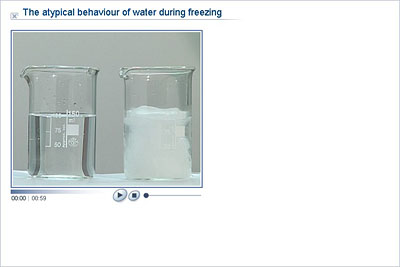The image appears to be a screen grab of a web page with a white background and a very thin light gray rectangular border. Inside this border, there is a caption at the top in dark blue text that reads "The Atypical Behavior of Water During Freezing," accompanied by a small gray 'X' on the left, indicative of a close button often seen in online content. Below this caption, there is a square visual element with a light blue outline, depicting two glass beakers on a white tabletop against a gray wall backdrop. The left beaker contains clear liquid water, while the right beaker shows partially formed ice with some remaining liquid at the edges. Below this visual, there are video controls suggesting the image might be an online video. These include a timeline marked from 00:00 to 00:52, a play button, a stop button, and a volume control slider. This detailed visual component emphasizes the different states of water during the freezing process, as indicated by the title.